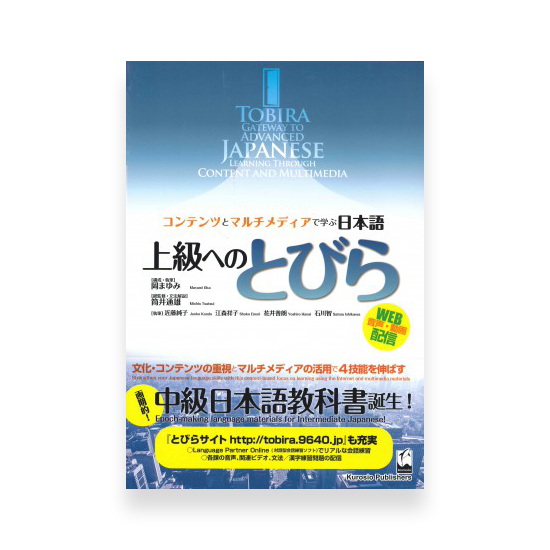The image appears to be a promotional poster, likely for a Japanese language learning program or resource titled "Tobira: Gateway to Advanced Japanese Learning Through Content and Multimedia." The background features a gradient that transitions from dark blue at the top to white in the middle, and then back to blue towards the bottom. Central to the image is the title text in English, rendered in white, descending from the top. This is accompanied by various Japanese text in both black and white colors.

A conspicuous illustration in the middle of the poster depicts a whitish-blue path leading to a slightly agile-looking, pale blue door. Below this illustration, the bottom section of the poster showcases a blue-tinted aerial view of a cityscape, complete with skyscrapers and buildings. 

Additional elements include a yellow circle on the right, which contains black Japanese text, presumably referring to a web address, and a large yellow banner stretching almost across the entire bottom of the image, also filled with black Japanese text. There are highlighted kanji characters in black on a yellow background interspersed throughout the advertisement, providing more detailed information, possibly including a website and contact number. The combination of text and imagery emphasizes the educational and multimedia focus of the "Tobira" program.